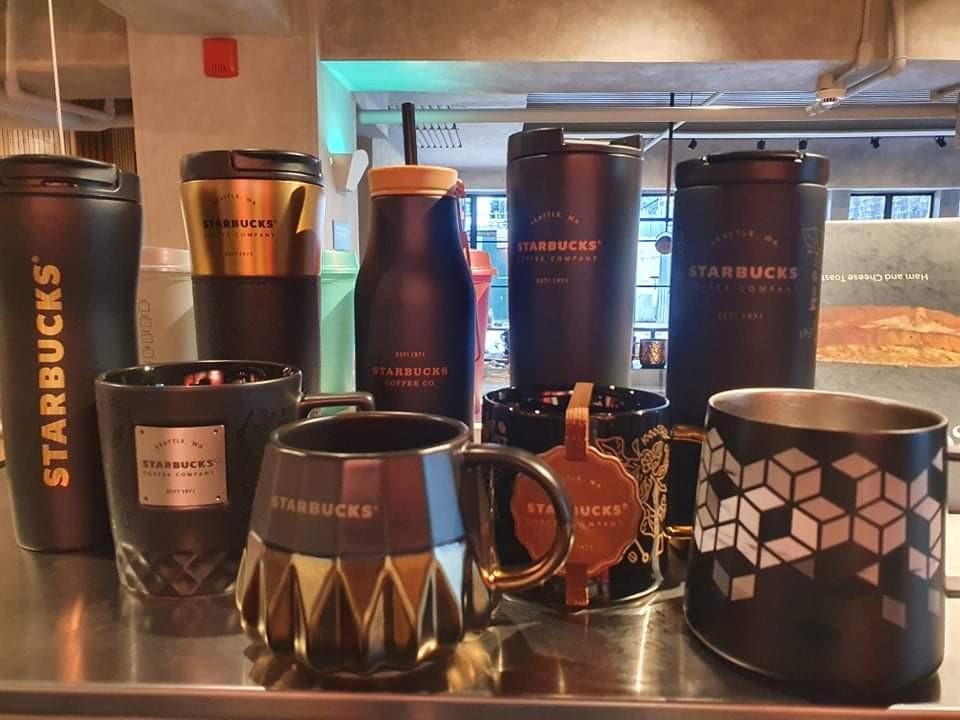This is a color photograph of a showcase display inside a Starbucks coffee shop, featuring an array of Starbucks-branded coffee cups and mugs on a stainless steel countertop. The background reveals an industrial or commercial setting with elements of gunmetal gray, stainless steel, and varying shades of tan, brown, and white, including some glass windows that provide a glimpse of the street outside. 

Front and center, there are two distinct lines of coffee containers—taller, cylindrical, insulated coffee cups in the back, and traditional coffee mugs with handles in the front. The tall cups primarily feature a black or green base with gold accents and are adorned with the Starbucks logo in silver or black fonts. Each has a unique design element: one has a gold reflective top, another mimics a milk jug with a gold cap and black straw, while others are plain cylindrical forms with flip-top lids.

The front row consists of varied coffee mugs, each decorated with unique patterns and textures. From left to right, one mug boasts a blue hue with white and gray diamond patterns, another is black with floral gold embroidery and a cardboard-like Starbucks tag, followed by a mug with a silver base and a gunmetal gray or black top with angular edges. Lastly, there's a green or black mug with a diamond-patterned base and a smooth circular top, emphasizing a central stainless steel logo plate of Starbucks branding.

All of these cups, primarily in tones of black and gold, reflect the standard and style the brand is known for, with designs emphasizing the Starbucks name.